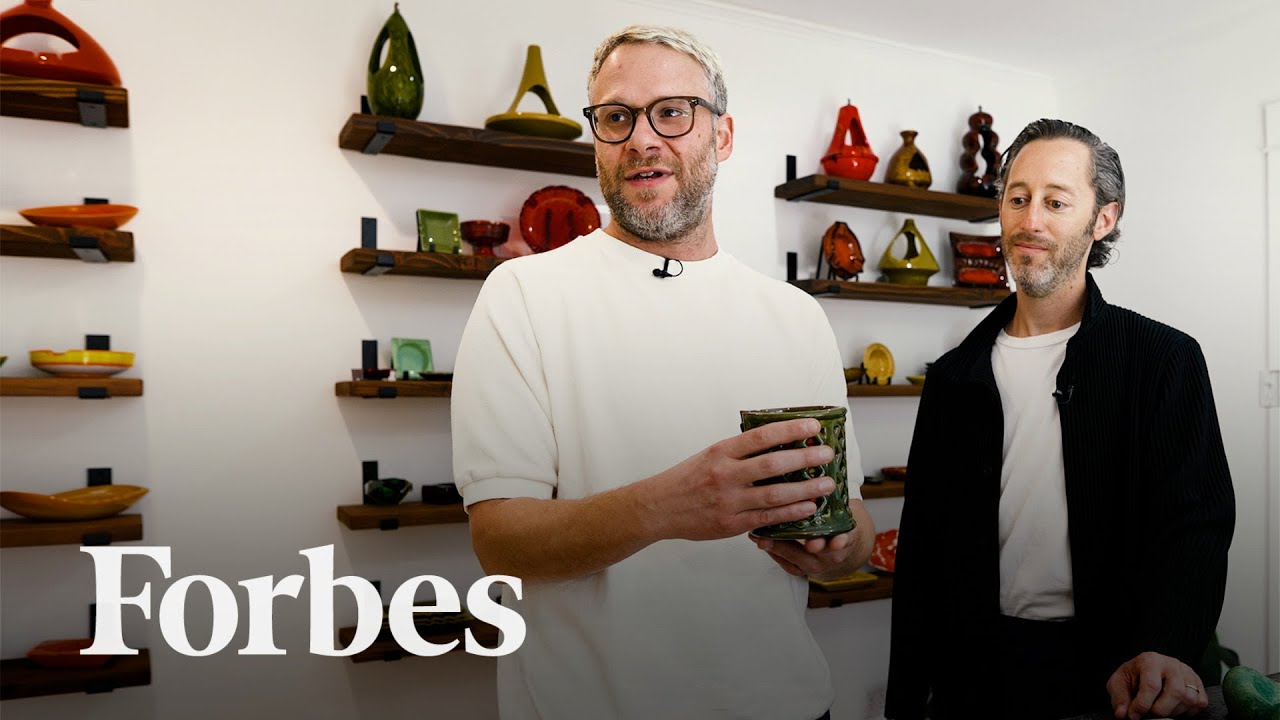In this close-up photograph, two men stand in a room with light gray walls and ceiling. The man in the center, identified as Seth Rogan, sports large black frame glasses, light blonde hair, and a graying full beard. He wears a white short-sleeved shirt with a clip-on black microphone on his left collar. Seth is holding an ornate green ceramic mug or pot at chest height with both hands—his left palm supporting the base and his right hand gripping the mug's side. To his right, another man with a graying beard and hair stands in a black jacket over a white undershirt and black pants. Both men focus their attention on the ceramic mug. The background features wooden shelves mounted on a white wall, displaying various ornamental objects, likely clay pots or tribal-like figures. In the bottom left corner of the image, “Forbes” is printed in white text.